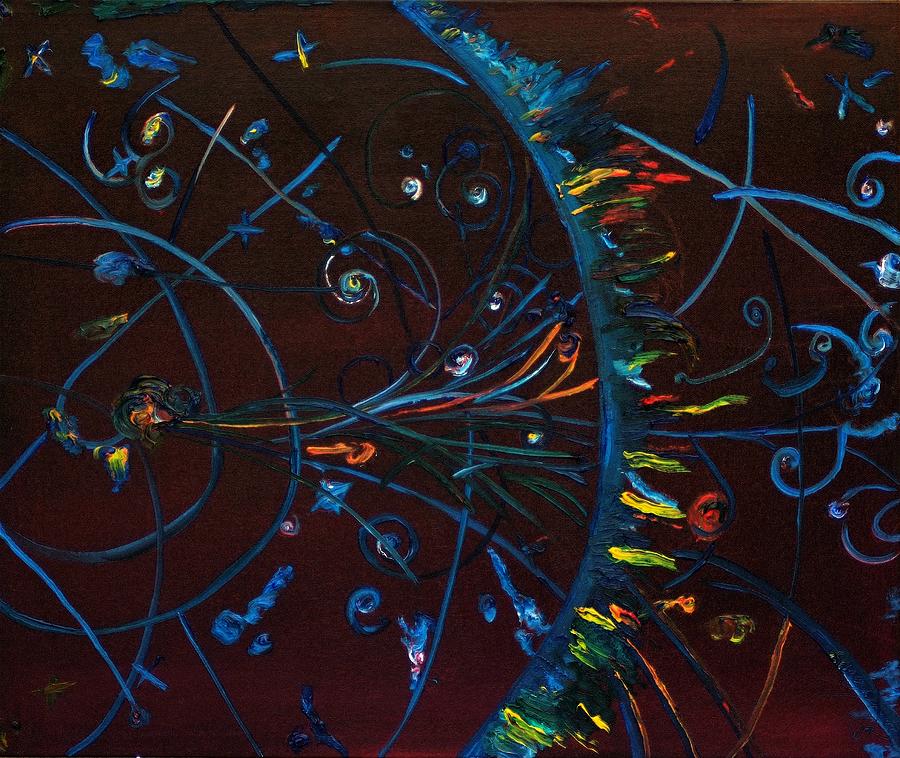In this vibrant abstract painting, the artist employs a dynamic interplay of colors and patterns to create a visually captivating piece. The foreground is dominated by a rich maroon-red that sets a bold tone for the artwork. Scattered across the canvas are multiple dashes of blue, which crisscross in string-like formations, adding depth and movement. A feather-like pattern intricately weaves through shades of yellow, turquoise, blue, red, and orange, creating a harmonious blend of warm and cool tones. The overall composition features predominantly upright elements, suggesting a sense of uplifting motion and energy.